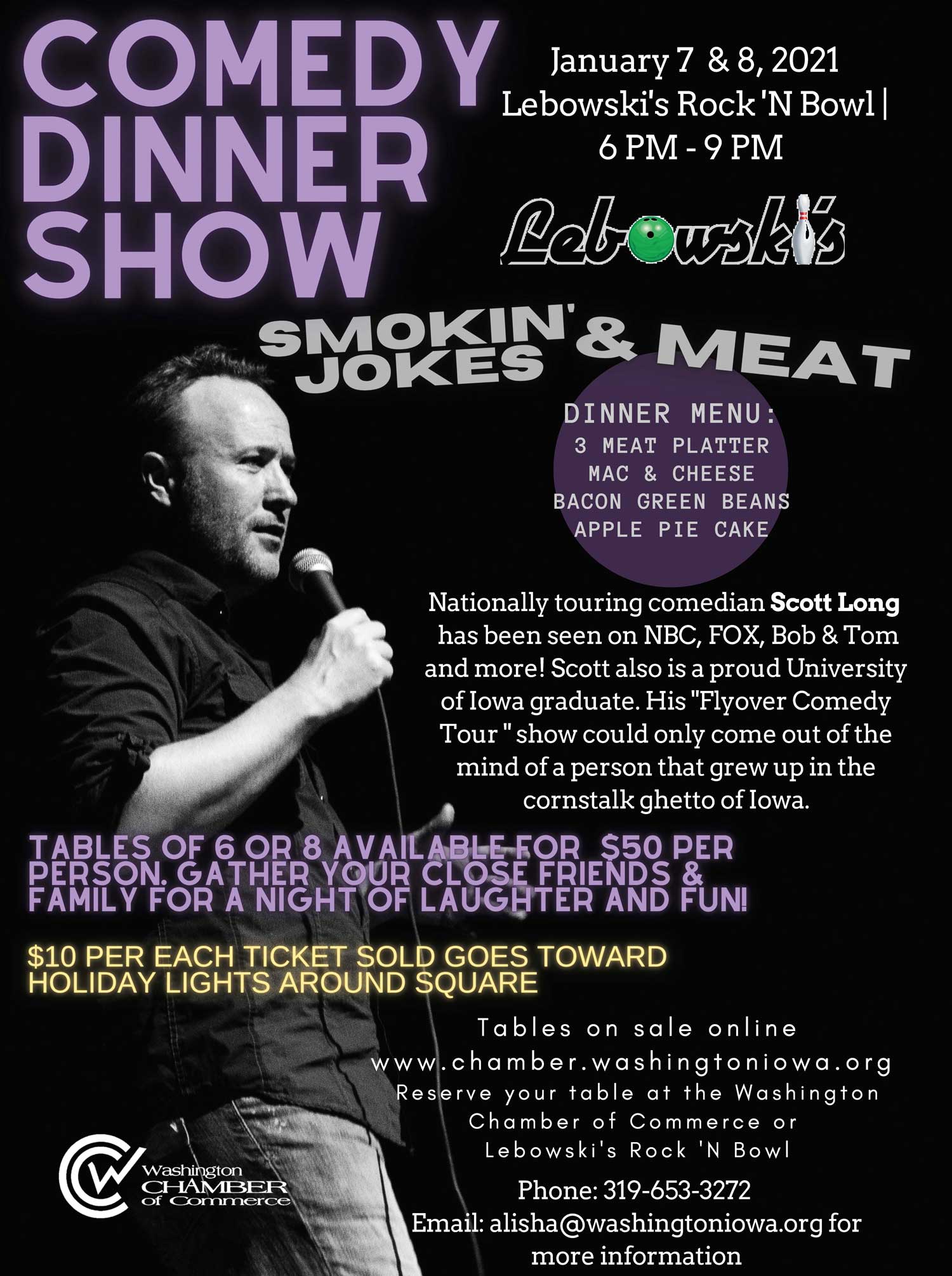Join us for a hilarious Comedy Dinner Show at Lebowski's Rock and Roll Bowl on January 7th and 8th, 2021, from 6 p.m. to 9 p.m. The event, aptly titled "Smoking, Jokes, and Meat," features standout comedian Scott Long, seen on NBC, Fox, and Bob and Tom, and a proud University of Iowa graduate known for his unique "flyover comedy." Enjoy a delectable dinner menu featuring a three-meat platter, mac and cheese, bacon, green beans, apple pie, and cake. Tickets are $10, with proceeds supporting Holiday Lights around the square. Reserve your tables of six or eight through the Washington Chamber of Commerce. Don’t miss out on this fun evening set against the backdrop of Lebowski’s bowling-themed venue!